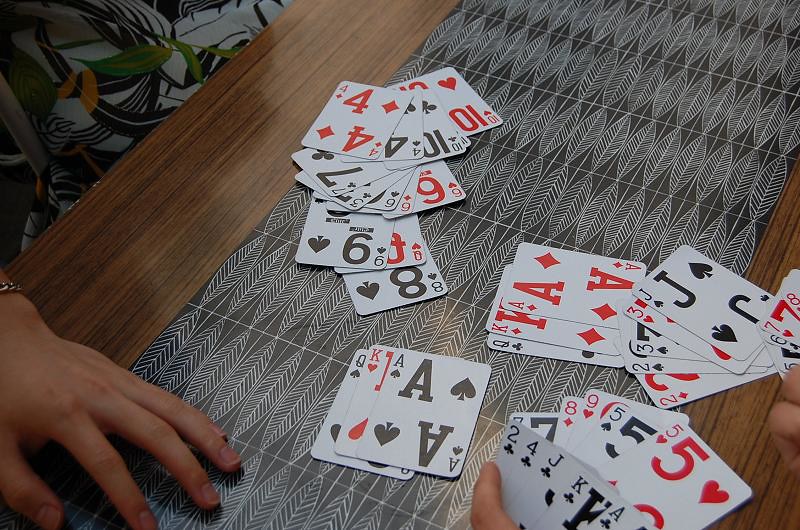This photograph features an array of oversized playing cards, each displaying large numbers and suit indicators, meticulously spread out on a coffee table-like surface. The table's surface is an illustrated wood grain, suggesting it is not real due to visible scratches, bumps, and bruises noted in the upper left section. In the background, a decorative cushion, likely belonging to a couch, can be seen, adding a homely touch to the scene. In the lower left corner, a left hand and wrist adorned with a gold-colored chain bracelet are partially visible, suggesting someone is about to participate in the card game. The playing cards belong to a standard deck, including jacks, kings, aces, and suits of hearts, diamonds, clubs, and spades. The distinctive large designations on each card make them stand out prominently against the simulated wood grain surface.